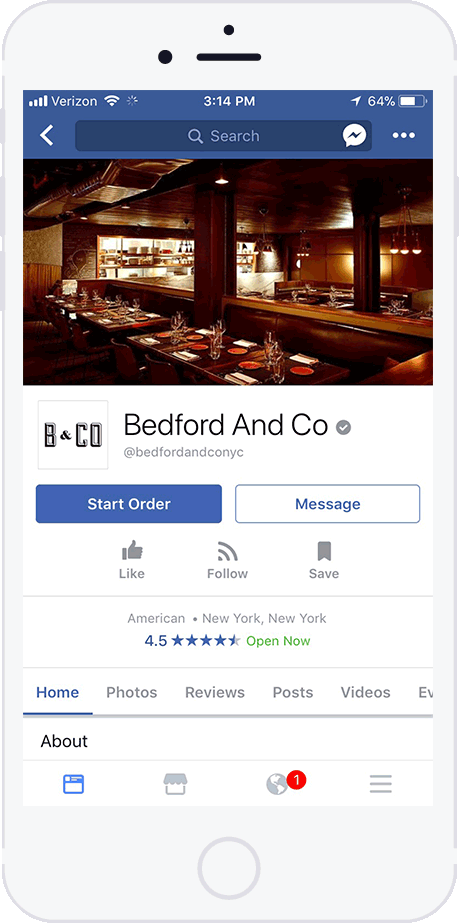The image displays a smartphone screen with a variety of elements and icons indicating it is currently on a restaurant's profile page within an app (likely a social media platform or restaurant review app). At the top, the status bar shows:

- **Indicators**: 
  - A 64% battery icon.
  - The current time, 3:14 PM.
  - The Verizon carrier name.
  - A Wi-Fi icon.

Below the status bar, there are navigation and search features:
- A back arrow pointing left.
- A dark blue search bar with a magnifying glass icon labeled "Search."

Next to the search bar:
- An icon resembling a speech bubble with a lightning bolt and three consecutive white dots.
- An image of what appears to be a restaurant.

Further below, the restaurant's details include:
- A partially visible area showing "BNCO" followed by "Bedford NCO."
- A small grey circle with a white checkmark inside.
- A website link beneath the name.

There are several blue and gray rectangles each labeled with different actions:
- A blue rectangle reading "Start Order."
- An outlined blue rectangle reading "Message."
- A thumbs-up symbol with the word "Like."
- A Wi-Fi-like symbol labeled "Follow."
- A bookmark icon labeled "Save."

Below these buttons, further information about the restaurant:
- The address area: "America dot New York, comma New York."
- A rating system showing 4.5 stars (4 completely blue stars and one partially blue, partially grey star).
- A green text label stating "Open Now."

Navigation tabs at the bottom include:
- "Home" in bold with a blue underline.
- "Photos," "Reviews," "Posts," "Videos" (with the last word partially cut off).

Further description includes additional buttons:
- A white rectangle labeled "About."
- An array of icons resembling a disc, a window, a planet, and a red circle with the number "1" inside of it, aligned vertically with three horizontal lines beneath.
- A large grey circle at the bottom of the screen as an additional navigation element.